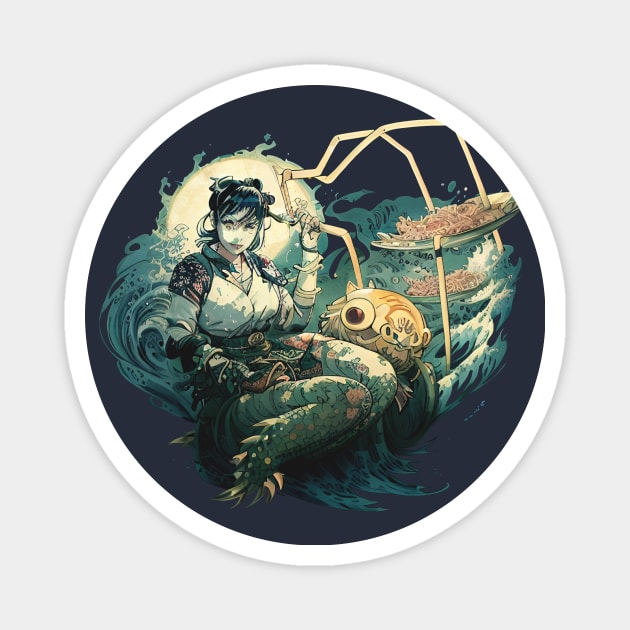This image is a circular, colorful drawing that appears to be in an anime style, set against a light gray background with a white border. At the center of the drawing is a young woman with long, dark, pinned-up hair, sitting cross-legged in a serene, underwater scene. Her facial skin is notably light, almost white, and her eyes are closed, exuding a calm and contemplative mood. She wears a distinctive, ancient-looking uniform primarily composed of green, white, and black colors. Her lower body forms into a scaly, mermaid-like tail.

In her left hand, she holds a golden, rod-like object with several arms or rows extending from it. Sitting or standing near her legs is a brown, round-shaped creature with bulgy eyes that resemble a mutated or animated fish. The scene is set against a dark blue background with curved waves of water, and a full moon glows behind the woman, adding to the magical and mystical atmosphere of the artwork.